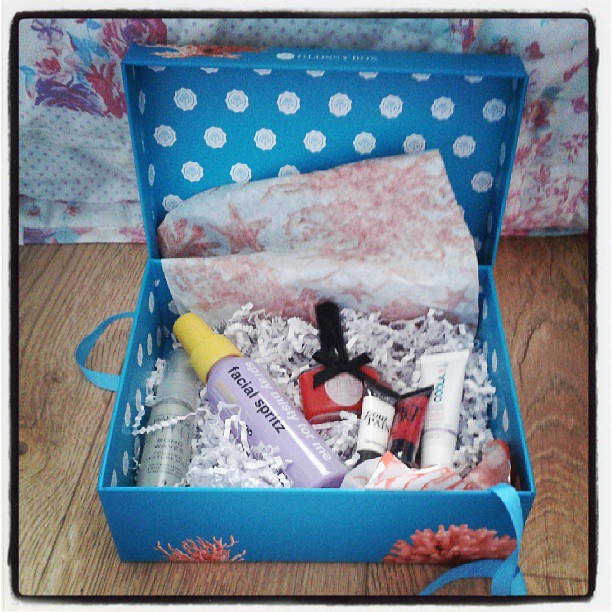The image portrays a boxed gift set filled with various beauty products, set against a backdrop of floral wrapping paper with shades of purple and pink visible in the top corners. The rectangular box is blue with white floral designs inside, and pink, almost coral-like decorations on the outside. It contains white tissue paper featuring pink stars and shredded white paper. Inside the box, there is a facial spritz labeled "Spray Misty for Me" in a light lavender bottle, a gray spray bottle, a red nail polish, and what appears to be a red lip gloss. Additionally, two small white tubes are included, likely samples of cream or lotion. The gift set rests on a wooden floor, leaning against what appears to be a floral sheet with hues of pink, white, blue, and purple. A thin black border frames the entire photograph.